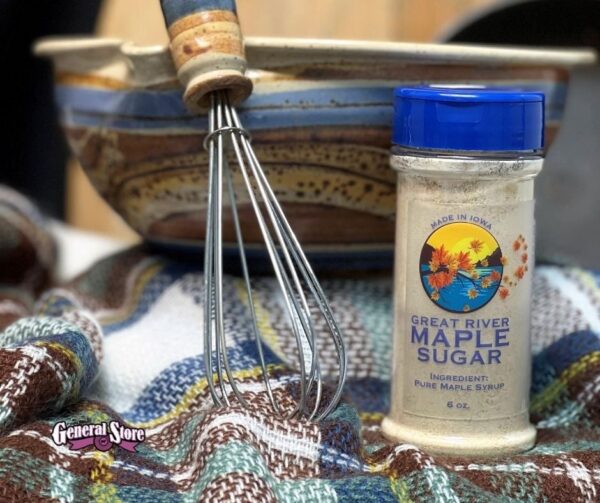The image features a check-patterned fabric in blue and yellow laid out at the base of the picture. On the right side of the fabric sits a small jar of Great River Maple Sugar, resembling a typical spice jar, with a label that includes depictions of maple leaves, a blue lake, and the phrase "Made in Iowa" in blue. The jar is topped with a blue lid. To the left, resting against a colorful mixing bowl adorned with blue stripes, brown tin, and brown speckles, is a whisk, the tines of which are placed flat on the fabric. Notably, the colors of the whisk and the bowl suggest they might be part of a set. Additionally, a white icon of a general store with a purple ribbon is located at the bottom left corner of the image. Overall, the scene suggests a kitchen setting with various warm and inviting tones, including blue, white, yellow, orange, brown, gray, and tan.